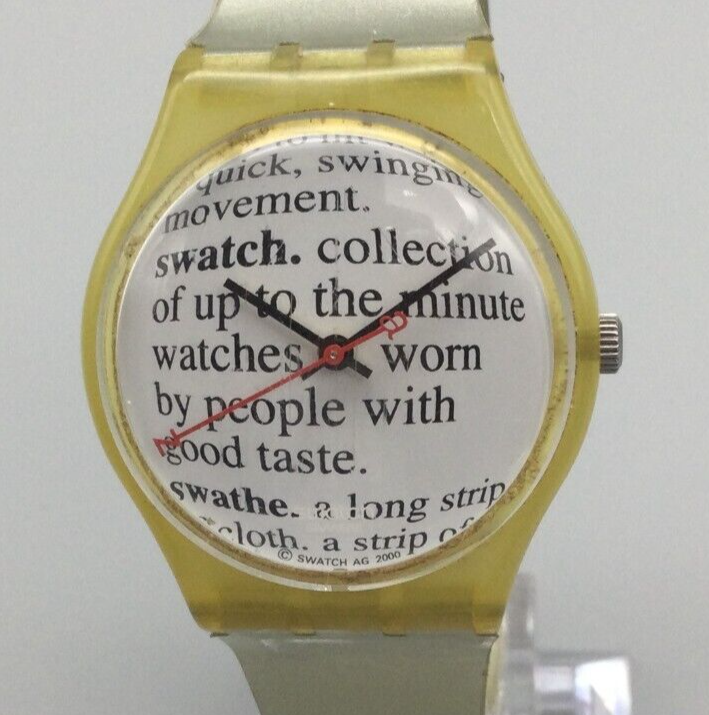This is a close-up photograph of a wristwatch centered on a light gray background. The wristwatch features a yellow, aged plastic body and cream-colored straps. The circular display screen shows the time at approximately 10:10. The minute and hour hands are black, while the second hand is red. Encircling the hands, black text is neatly arranged against a white backdrop. The text reads, "Quick swinging movement. Swatch collection. Up-to-the-minute watches worn by people with good taste." Additionally, the word "swatch" appears in bold, followed by "a long strip of cloth," giving a dictionary-like definition. The overall composition focuses on the detailed elements of the watch's face, highlighting both the stylish design and the intricate text.